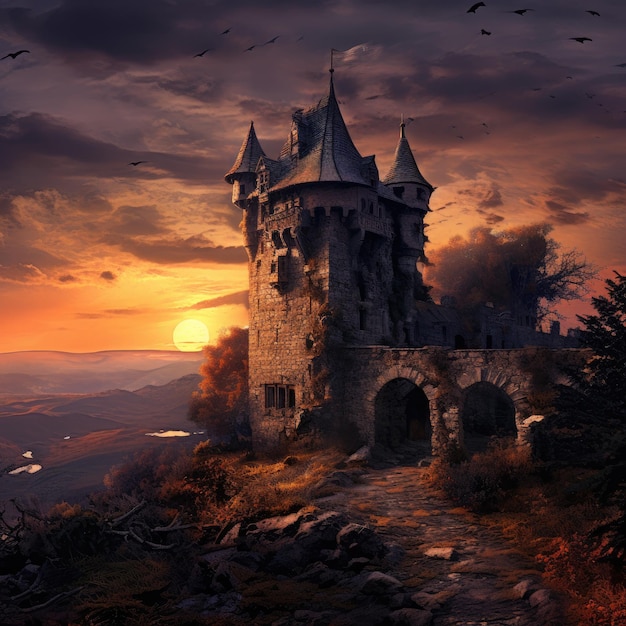This detailed painting depicts a weathered, old castle situated at the edge of a rocky cliff, commanding the majority of the foreground, particularly the right and lower sections of the image. The castle features a large, sturdy central tower with a conical roof on the left side, and a wall with two arched entryways extending to the right. Several round turrets rise from the top of the castle. In front of the castle, the ground is dotted with trees, shrubs, and rocky terrain.

In the background, the valley opens up beneath sloping mountains and hills, interspersed with glimmering lakes reflecting the setting sun. The sun, hovering just over the horizon, casts a warm, golden glow across the landscape, transitioning the sky from deep purplish-gray at the top to a bright orangish-yellow near the horizon. Birds are scattered across the cloudy sky, adding life to the serene scene. The overall atmosphere suggests the close of day with an impending twilight that adds an enchanting aura to the medieval castle scene.